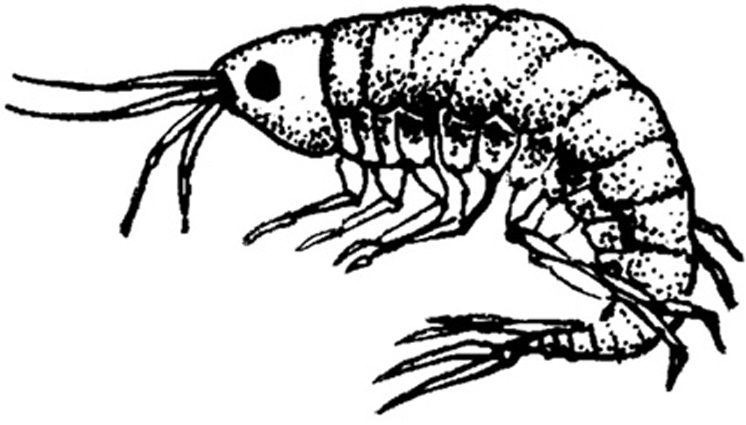The image is a black and white sketch of a crustacean, possibly a crawfish or shrimp, set against a plain white background. This detailed drawing reveals various anatomical features of the creature. The head prominently features four protrusions emerging from its mouth area and a dark, solid black eye. The body is segmented, consisting of a total of thirteen parts, with nine larger segments leading into smaller segments towards the tail end. The crustacean has multiple legs, with at least four towards the front on each side and additional ones towards the back, totaling around eight visible legs. The tail tapers into three distinct prongs. The entire sketch appears to use dotted textures to highlight certain features, adding depth to the black outlines. There is no accompanying text in the image.